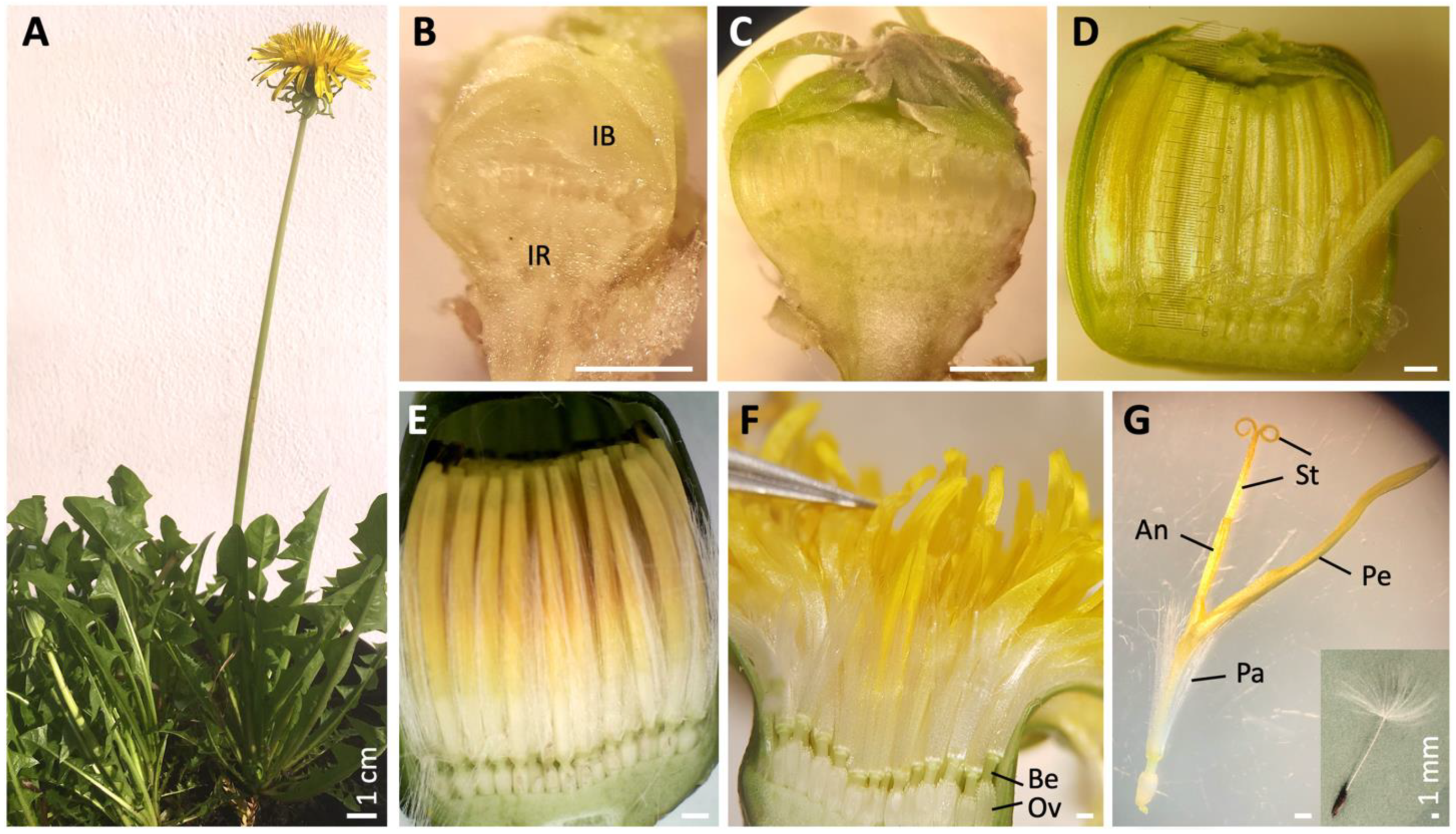The image showcases a detailed, labeled progression of a dandelion flower's development, starting from the left and moving to the right through seven stages labeled A through G. On the far left (A), the dandelion with its vibrant green leaves sits against a white background, with a long stem and a yellow flower at the top. Moving to the right, stage B features a translucent yellow bud. In stage C, the bud appears darker and starts opening. Stage D shows a greener bud beginning to split, revealing some yellow. By stage E, the flower opens more, displaying yellow shoots. In stage F, the flower is almost fully open, prominently yellow. Finally, in stage G, various dissected parts of the flower are shown for size comparison, including a small piece of white dandelion fluff, indicated to be approximately one millimeter.